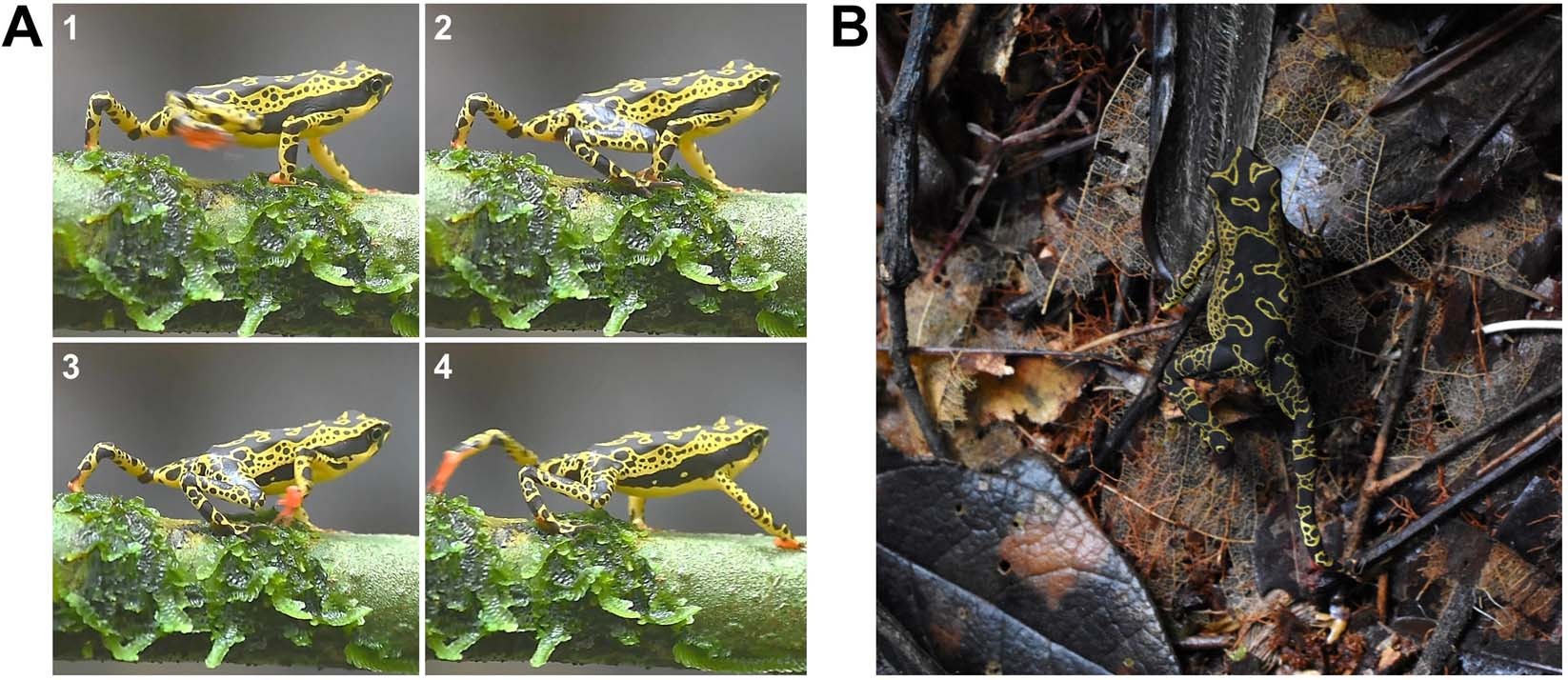The two-part image features frogs labeled A and B, designed for a detailed description that might be found in a science book. Image A, on the left, is a progression strip split into four individual boxes labeled 1, 2, 3, and 4, depicting the same frog walking on a branch. The frog, yellow with black stripes and dots and possessing a red underbelly and red feet, shows various stages of movement with its elongated legs as it moves past the green part of the branch. Image B, on the right, captures a single large black frog with yellow, tiger-like stripes and intricate circle patterns on its back. This frog is seen with its right leg extended, walking on a forest floor strewn with dried leaves and pine needles, set against a dark background.